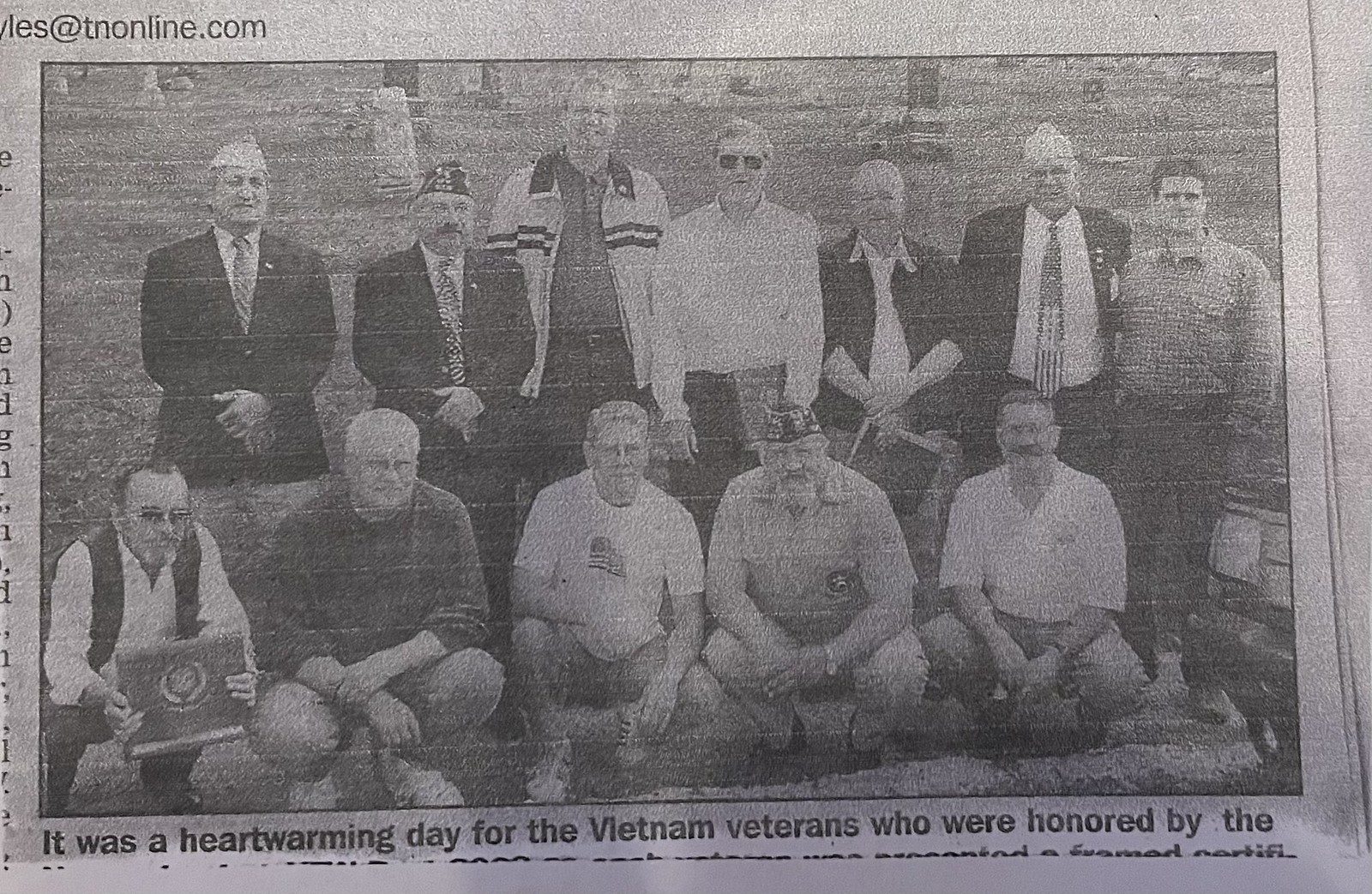The black-and-white image is a faded, aged newspaper clipping. The photograph, which occupies most of the clipping, features a group of Vietnam veterans. Seven men are standing in the back row, while five men are kneeling in the front. Several of the men are wearing suits and ties, with some donning their military hats adorned with awards and pins. A few men are holding plaques with awards, and one man is holding a small American flag. The veterans appear to be in a cemetery or a memorial garden, and most are smiling at the camera. The caption beneath the photo reads, "It was a heartwarming day for the Vietnam veterans who were honored by," with the remaining text cut off and unreadable.